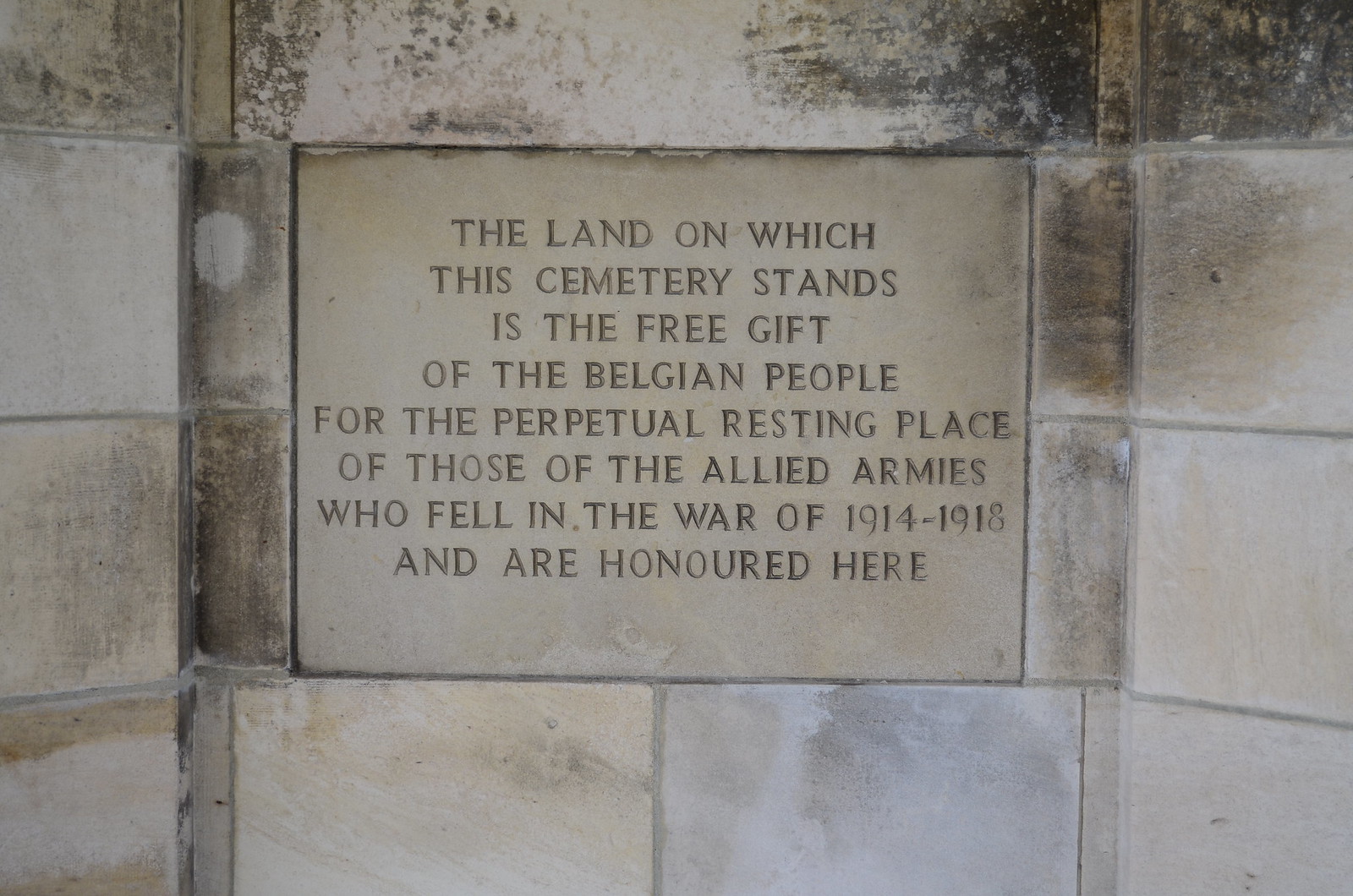The image features a rectangular stone wall composed of large, weathered blocks of marble, with noticeable discoloration ranging from brown to dark black towards the top and newer, cleaner stones towards the bottom. Mortar is clearly visible between each block, giving the wall a historic appearance. Centrally embedded in this wall is a large tan stone plaque, roughly two blocks high and two blocks wide. The plaque is meticulously inscribed with the words: "The land on which the cemetery stands is the free gift of the Belgian people for the perpetual resting place of those of the Allied armies who fell in the war of 1914 to 1918 and are honoured here," noting the British spelling of "honoured." This engraving indicates that the site is a war cemetery dedicated to soldiers from World War I, spanning the years 1914 to 1918.